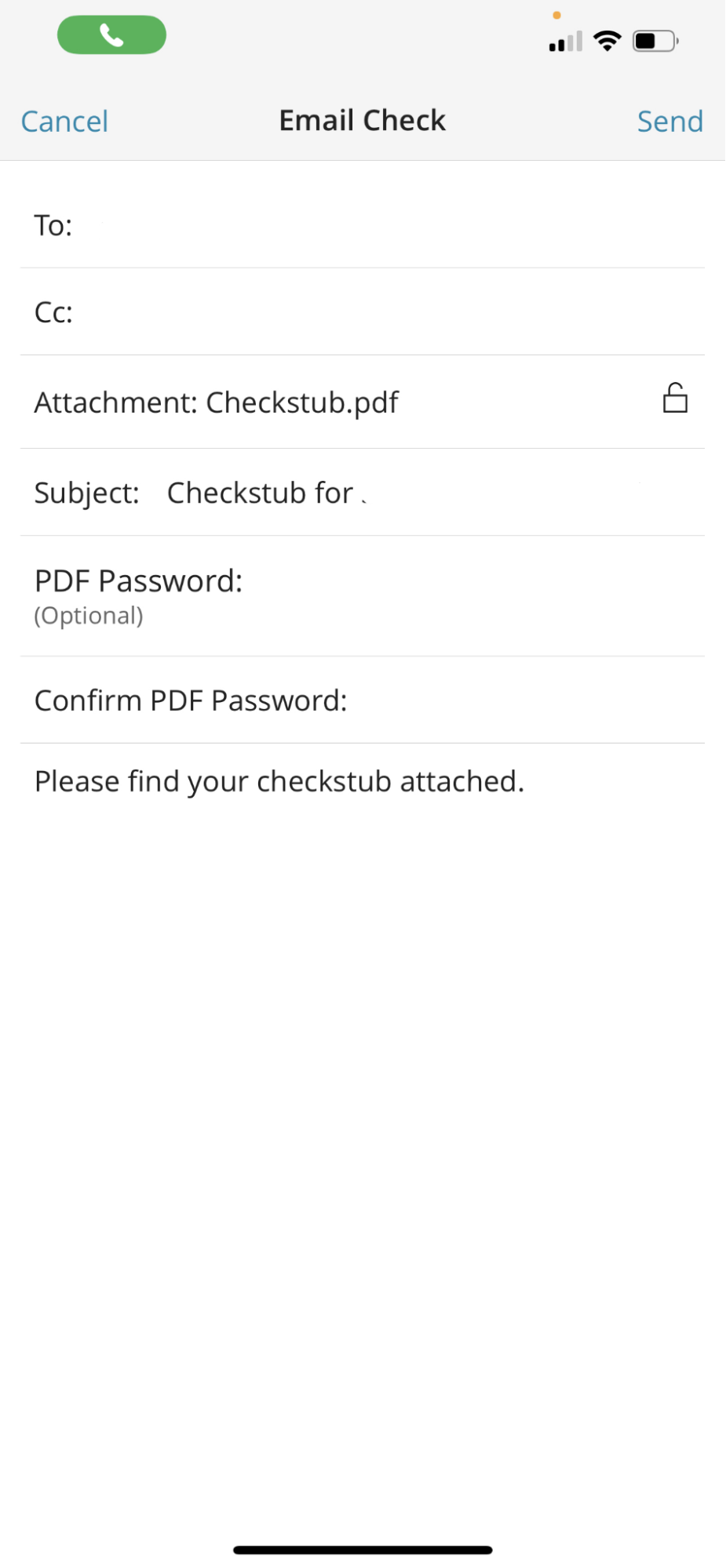The image is a screenshot taken from a cell phone. At the very top of the screenshot, there is a pale grey bar spanning the width of the device. On the left side within this grey bar, a green capsule icon containing a white phone symbol indicates an active call. On the right side of the grey bar, icons indicate signal strength, Wi-Fi connectivity, and battery level.

Immediately below this grey bar, a smaller section contains three key options: "Cancel" on the left, "Email Check" in the center, and "Send" in blue on the right.

The subsequent content below these options is positioned against a predominantly white background. The first line is labeled "To," but it remains empty. The line below it is designated for "Cc," which is also unfilled. Following that, there is a line labeled "Attachment" that includes a file named "checkstub.pdf," accompanied by an open padlock symbol on the far right.

Next, the "Subject" line reads "checkstub4." Underneath the subject line, there are fields for "PDF Password" and "Confirm PDF Password," both of which are marked as optional. The body of the email contains the text: "Please find your checkstub attached."

Lastly, at the very bottom of the screenshot, there is a short black line indicating navigation options, suggesting that swiping up will close the screen or swiping left to right will allow scrolling between windows.